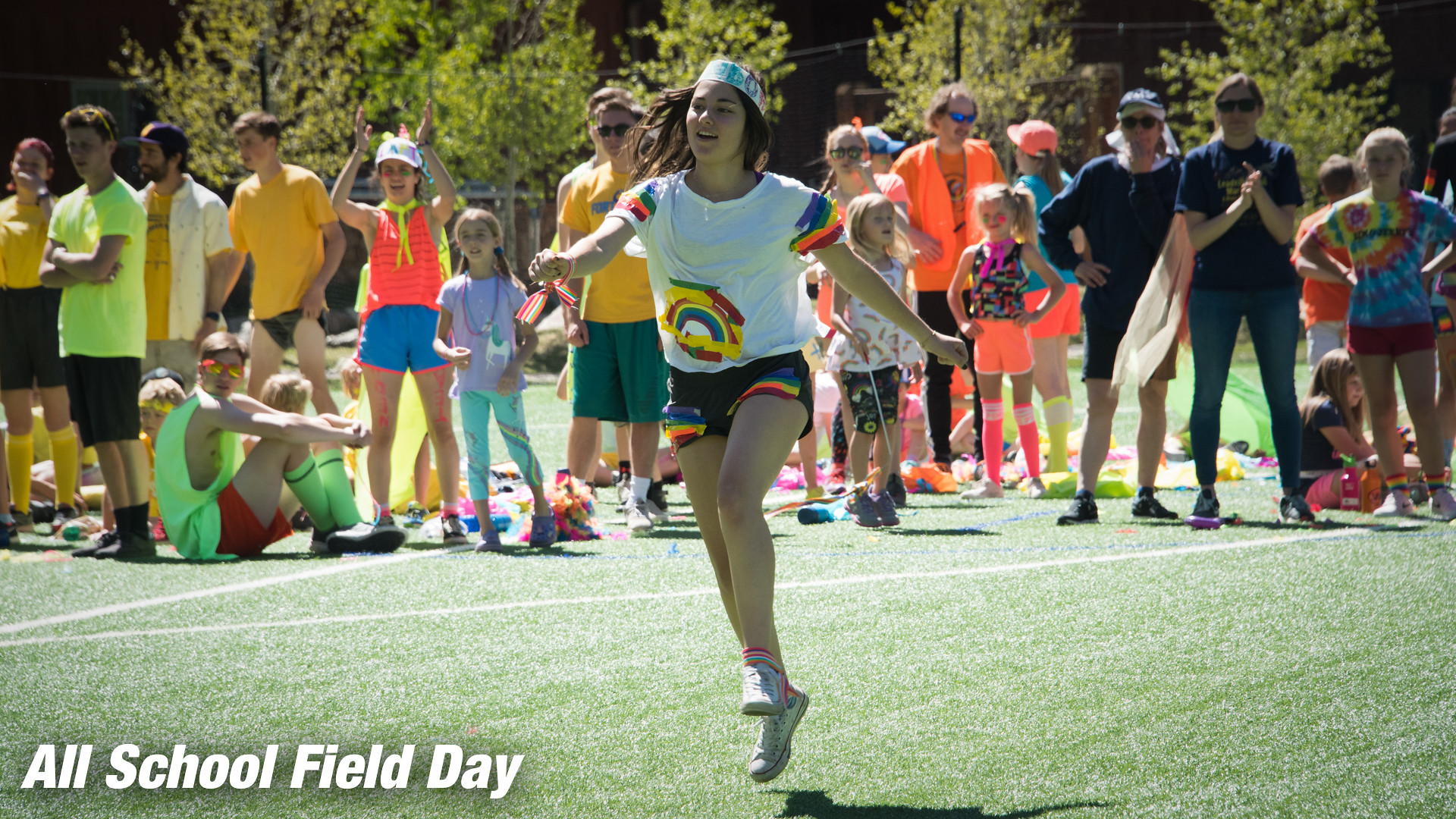The image captures a vibrant outdoor scene on a bright, sunny day during an All School Field Day event. It is set on a grassy field marked with white lines and surrounded by trees in the background. In the center of the photo, closest to the camera, is a young girl or teenager with long black hair, wearing a playful outfit consisting of shorts with a rainbow print, a white T-shirt adorned with colorful rainbow designs made from tape, and a makeshift paper crown on her head. She sports a wristband and white Converse shoes. The girl appears to be running or jumping, her hair flowing on either side. Behind her, a group of spectators, including both adults and children, are all facing the same direction, dressed in bright, varied colors, and either standing or sitting as they watch the event. In the bottom left corner of the image, white block letters spell out "All School Field Day."